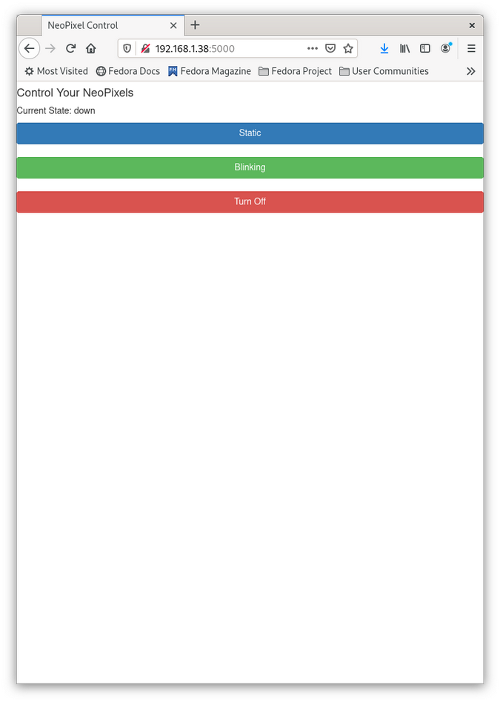In this image, captured from a computer screen, an open browser tab labeled "NeoPixel Control" is visible at the top. The tab title features the word "NeoPixel" written with a capital 'N' and 'P', followed by the word "control" in lowercase. Below this, a browser interface is shown, featuring standard icons like the home icon and a search bar. Beneath these icons, a list of categories appears, each prefaced by icons to their left, including "Most visited," "Fedora Docs," "Fedora Magazine," "Fedora Project," and "User Communities."

Centered below the top section, there is black text displaying "Control your NeoPixels," followed by a status indicator reading "Current state: Down." Further down, the screen is divided into three horizontal, rectangular sections that span the width of the viewable area. The first section is medium blue and contains the white text "Static" at its center. The second section is medium bright green, also centered with white text that appears to read "Blinking." The third section is red and bears the centered white text "Turn Off." These sections seem to represent different control options for managing NeoPixel states.